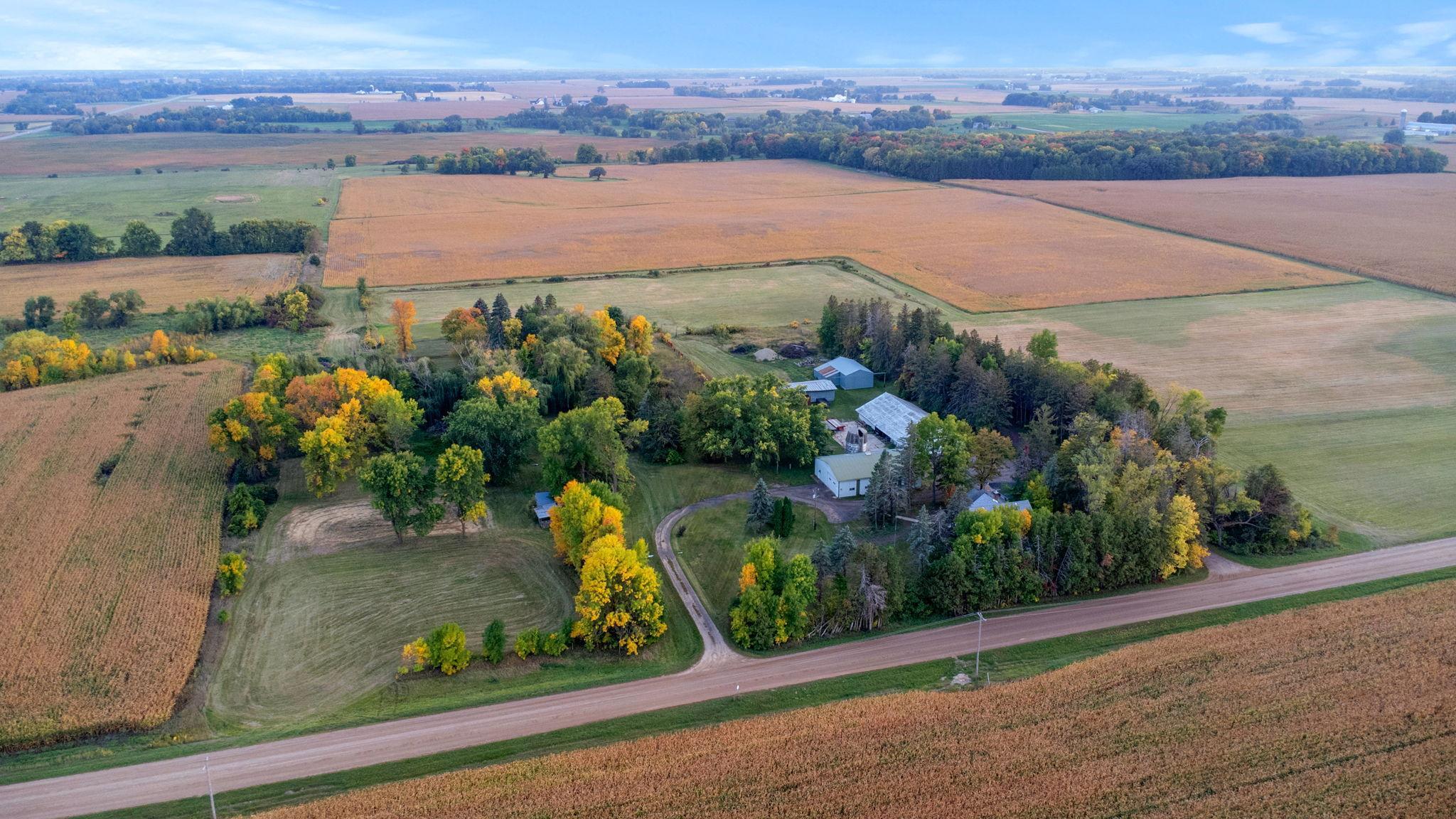An aerial photograph showcases a sprawling landscape of farmland, characterized by rectangular and square plots in varying shades of green and brown, the latter likely indicating either dry or harvested crops. A central wooded section draws attention with its cluster of green and yellowing trees, suggesting the image was taken during the fall season. Nestled amidst these trees are four white structures, possibly houses and barns, connected by a smaller dirt road extending from a main road that runs horizontally across the bottom of the image. Further in the distance, additional farmlands and a few more buildings are visible, hinting at a small rural town typical of the Midwest or the South. The sky above is a clear blue, dotted with wispy white clouds, completing this serene rural scene.